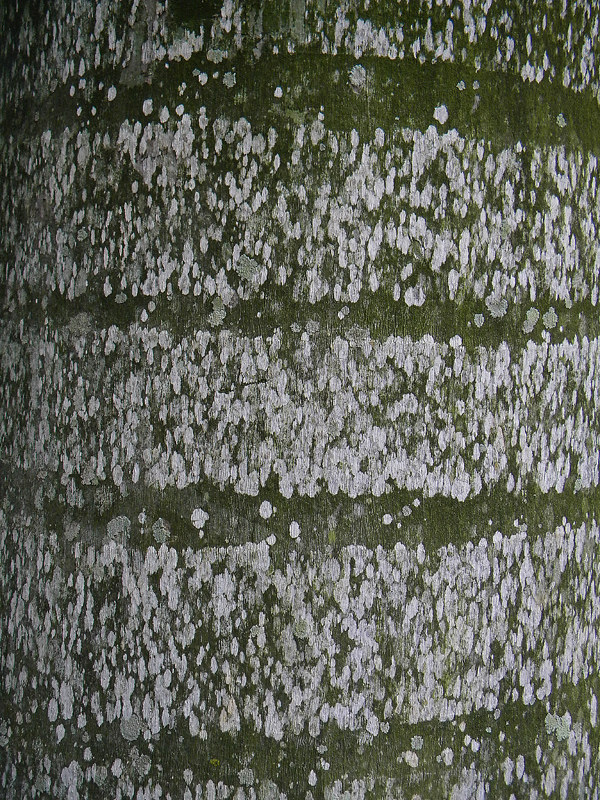This image appears to be a detailed piece of artwork, capturing an intricate close-up view of a scene evocative of natural elements. The background is predominantly a darker tree or pine green, with an overlay of white texture suggestive of snow. This green, rich in tone, provides a striking contrast to the off-white, snow-like patches, giving the canvas a compelling visual depth. The white texture is meticulously applied, possibly indicating fallen snow on a green surface, drawing parallels to a close-up view of snow-covered grass or a tree trunk.

The artwork also features a series of horizontal lines, four in total, creating a repeating pattern that enhances the sense of structure and rhythm within the piece. These lines could hint at the idea of straps once having been wrapped around a tree, as every six inches a segment of the green background is intersected, reminiscent of missing bark, which further emphasizes the painting's natural motifs.

The pattern is so precise and deliberate that it strongly suggests the image is a carefully crafted painting rather than a photograph. The green-gray hues in between the white lines add texture and depth, resembling moist, rain-kissed surfaces. This combination of colors and textures, along with the methodical arrangement, intricately blends the realism of natural elements with the abstract precision of artistic technique.